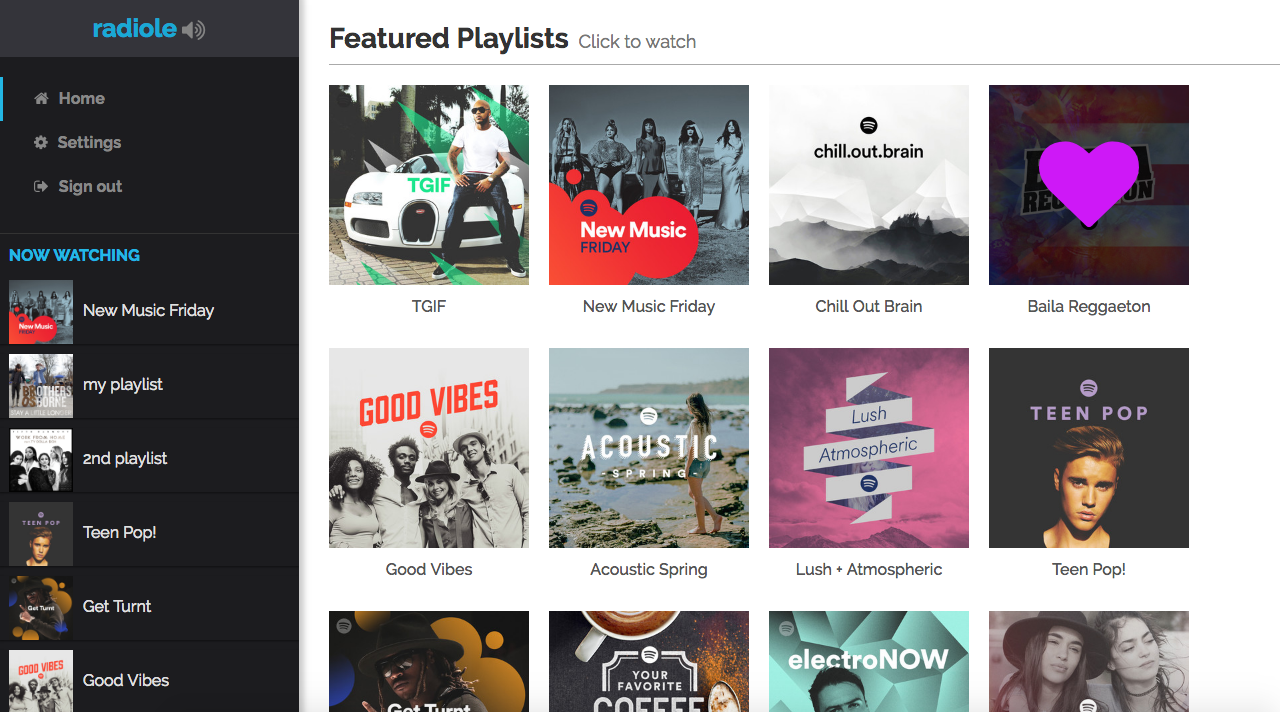The screenshot captures the interface of a music streaming service called "Radiole," as indicated by the bold text in the top left corner. The navigation bar at the top, displayed in a black header, includes options such as Home, Settings, Sign Out, Now Watch, New Music Friday, My Playlist, Second Playlist, Teen Pop, Get Turnt, and Good Vibes, accompanied by six album cover thumbnails beside each category.

To the right, the content section of the site is featured, showcasing several playlists categorized under "Featured Playlists" with a clickable option to watch. The titles of the playlists are TGIF, New Music Friday, Chill Out Brain, Bala, Reggaeton, Good Vibes, Acoustic Spring, Lush Atmospheric, Teen Pop, and four other unreadable titles. Each playlist is visually represented with a thumbnail or album cover: TGIF features an image of a man sitting in front of a car, New Music Friday displays a group of singers, and Teen Pop depicts a pop star. The background is predominantly white, with no other discernible elements visible in the image.